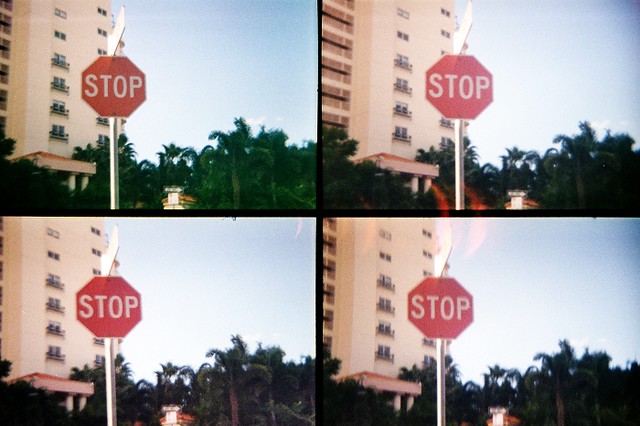This art piece features a collage of four nearly identical photographs of a stop sign arranged in a two-by-two grid. The stop sign, prominently displayed slightly left of center in each photo, is red with white block lettering and an octagonal shape, mounted on a tall silver metal post. A rectangular, glare-obscured street sign sits above the stop sign. Each photo is bordered by a thin black border, with the central dividing lines forming a cross-like structure in the middle.

In the background of all four images, the left half showcases a large tan-colored building, possibly a hotel or an apartment complex, with multiple small windows. The top-left photo reveals a portion of a balcony and two sets of windows, while the top-right photo shows the entire balcony along with the windows. The bottom-left photo displays just the two sets of windows, and the bottom-right photo includes a slightly larger section of the balcony than in the top-left but less than in the top-right image.

Behind the stop sign, on the right side of each photograph, there's a clear blue sky and numerous palm trees, with the upper-left image featuring a brighter green hue on the trees compared to the others.